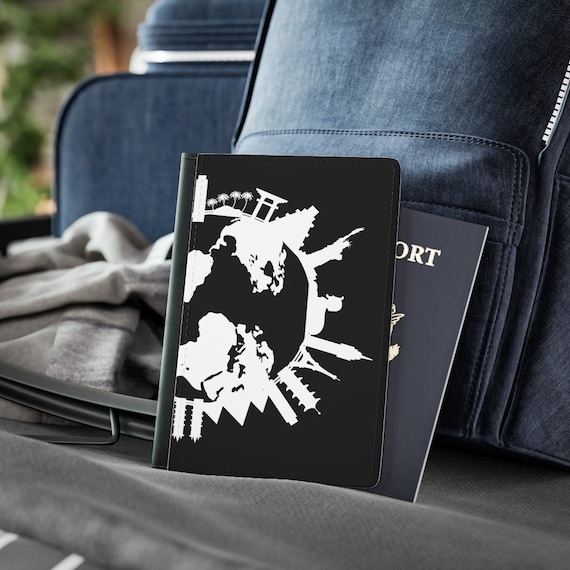A photograph taken inside a vehicle, likely the back of a bus due to the large window visible in the background. In the center of the image is a black and white notebook featuring a semi-circle design that depicts Earth, highlighting North America, South America, Africa, and Western Europe, with various city buildings around the globe design. The notebook is in a portrait layout, leaning against other items. Partially obscured behind the notebook is a smaller booklet, identified as a passport by the visible letters "ORT" and part of the seal. These items are resting against a black backpack and perched on a gray blanket. The lower portions of the scene show a lighter gray blanket off to the left, suggestive of passenger comfort on a bus. In the background, there is additional luggage and a blue seat. Through the window, greenery and foliage hint at a natural setting outside. The scene is devoid of people, with a primary focus on the travel essentials—passport, notebook, and luggage—arranged on the cozy fabric backdrop.